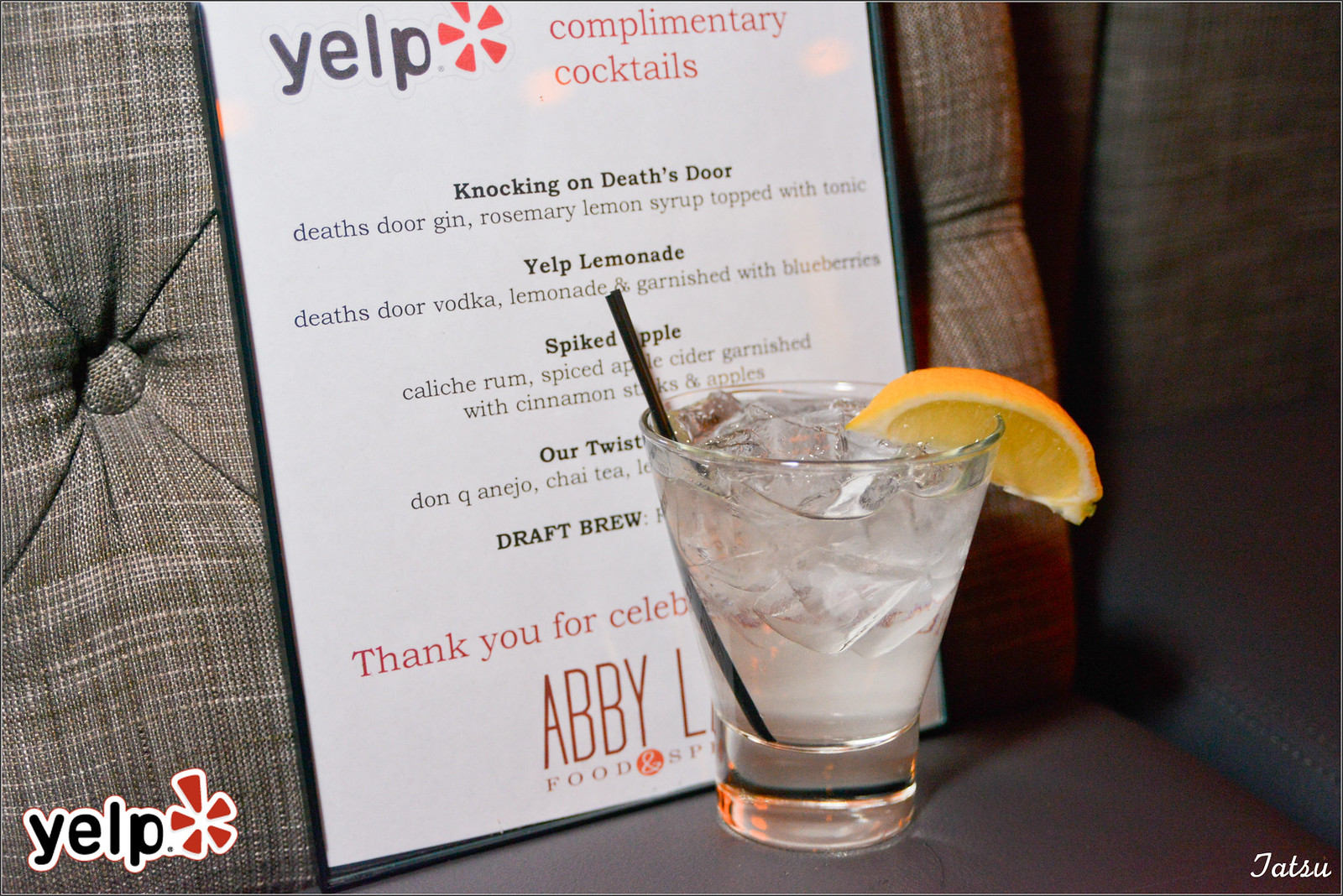This photograph, likely taken inside a bar or restaurant, captures an elegant cocktail scene. The centerpiece is a clear, ice-filled cocktail garnished with an orange wedge on the rim and a black straw. The drink, with its foggy clear liquid, sits to the right of center on a brown and gray plaid cushion, which appears to be part of a seat or bar booth. 

Leaning against the cushion is a distinctively bordered cocktail menu with a white background and black trim. At the top left of the menu, the familiar Yelp logo, featuring black lettering with a red flower symbol, stands out. Next to it, the words "complimentary cocktails" are prominently displayed. The menu lists several enticing options:
1. "Knocking on Death's Door" - a drink made with Death's Door Gin, rosemary, lemon syrup, and tonic.
2. "Yelp Lemonade" - featuring Death's Door Vodka and lemonade, garnished with blueberries.
3. "Spiked Apple" - partially obscured but indicating ingredients like Caliche Rum and spiced apple with cinnamon sticks.

The bottom of the menu includes more text, slightly obscured by the cocktail glass, with a note suggesting a celebration for Abby Ale or Abbey Labs, possibly a thank-you message from Yelp. 

Completing the scene, the lower corners of the image feature additional branding: the Yelp logo in the bottom left and "Tatsu" written in white cursive on the bottom right.